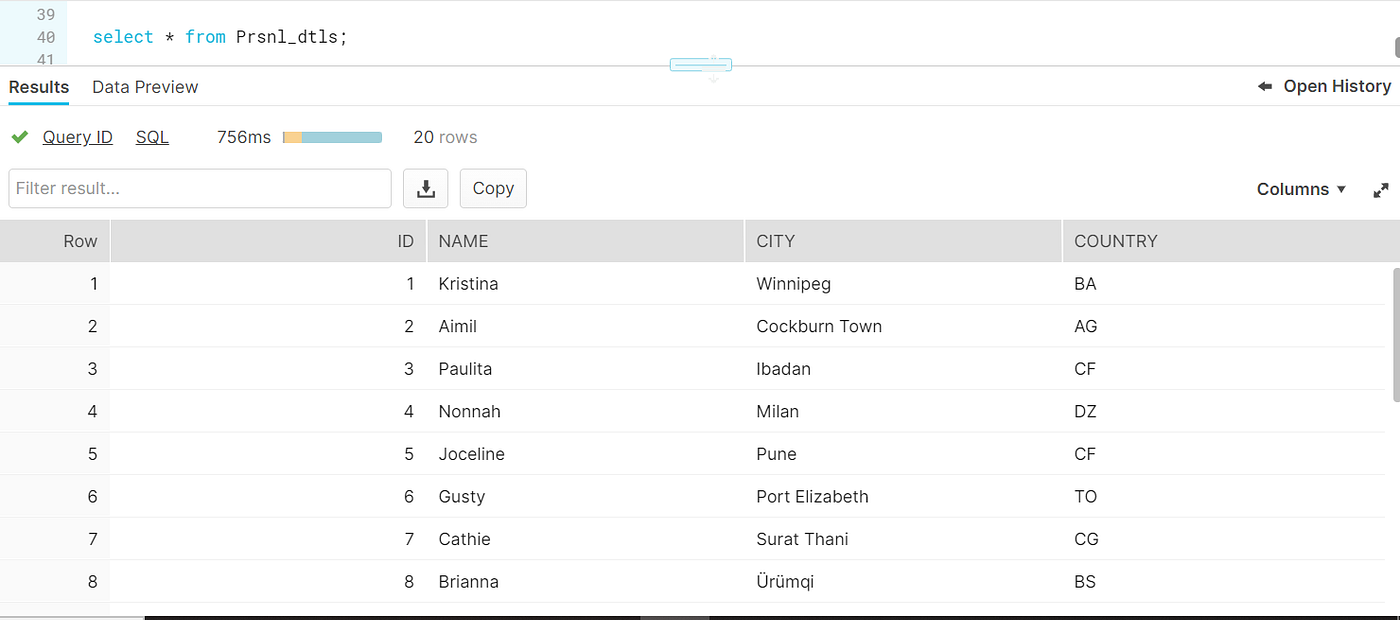This is a detailed photo capturing a computer screen displaying an online data interface. The screen has a white background, topped with a bar featuring numerical indicators "39," "40," and "41." To the right of these numbers, the text "SELECT * FROM PRSN1_DTLS" is visible. Directly below this, in black lettering, it reads "Results: Data Preview," and to the right, there is an "Open History" button with an arrow pointing left.

Further down, the text "Query ID SQL: 756 MS" appears above a bar that is partially orange and predominantly light blue, labeled "20 rows." Below this bar, a search box marked "Filter Results" is available, with options to download or copy the data situated to its right.

The main data table is displayed on a periwinkle background with black lettering, organized into five categories: "Row Number," "ID Number," "Name," "City," and "Country." Over the "Country" column, there is a drop-down menu titled "Columns" with an arrow indicating towards the lower left and upper right corners. Each of the eight rows in the table contains detailed sets of information relevant to these categories.